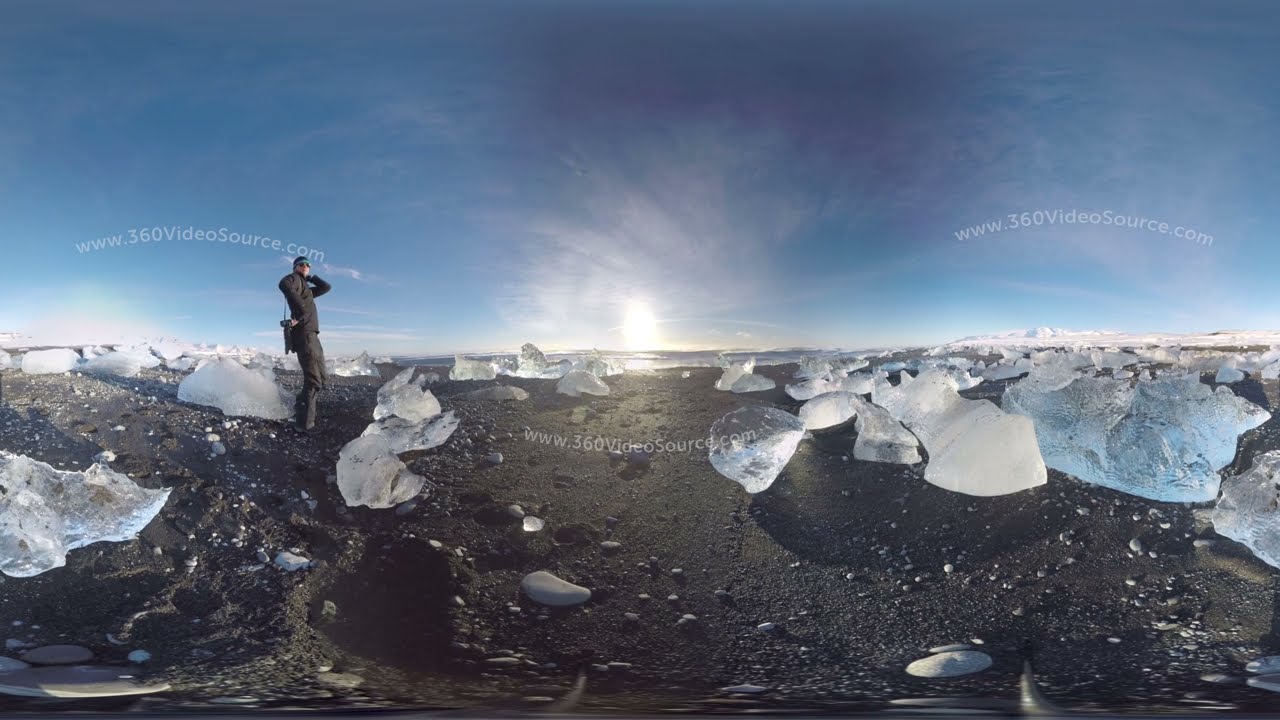This is an unusual and highly detailed rectangular horizontal photograph, likely captured with a special 360-degree lens, resulting in a noticeably curved and distorted image. The upper half of the composition features a very dark blue sky dotted with glowing white lights and a few scattered, high-altitude clouds. Dominating the center is the horizon line with a noticeable sun hotspot. The entire image is marked thrice with the text “www.360videosource.com,” gently curved, appearing in the upper left, center middle, and upper right corners. 

The lower half consists of a stark, bare ground that appears to be covered with snow or sand and dotted with massive, irregularly shaped ice boulders, suggesting an arctic or glacial terrain. The left third of the photograph captures a photographer wearing dark clothing, including a black beanie with a blue headband, crouching as if taking a picture. The right side of the image primarily contains these curved snow or ice formations with no identifiable buildings, contrasting with a faint and distant white building visible in the background on the left. The overall composition conveys a surreal, almost otherworldly landscape, intensified by the curvature and distortions of the 360-degree view.